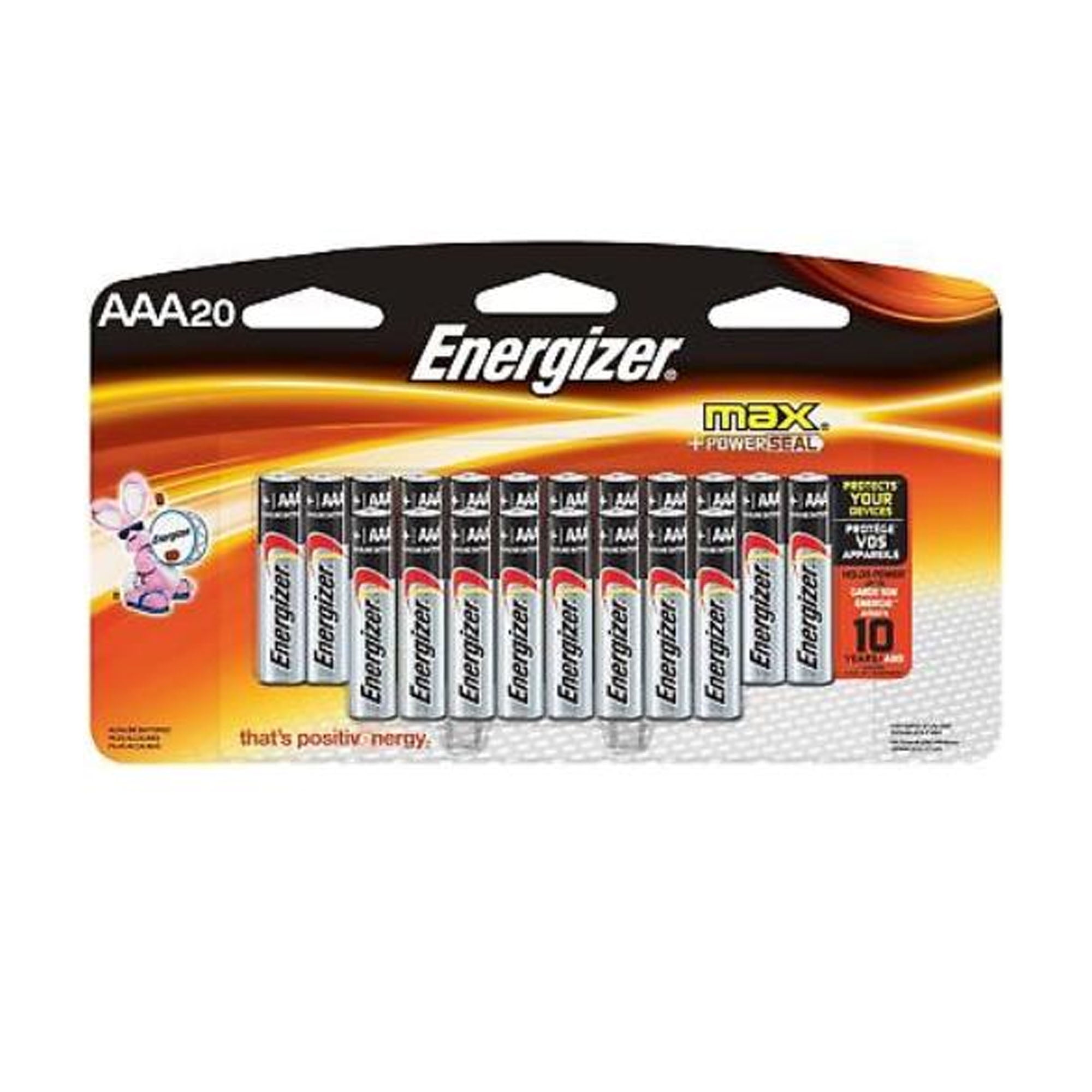Screenshot of a package of Energizer AAA batteries. The package contains 20 Energizer batteries and prominently features the iconic Energizer Bunny holding a drum with a drumstick. The text "Positivenergy" is displayed on the packaging, with "Positive" spelled as "P-O-S-I-T-I" and "Energy" spelled as "N-E-R-G-Y." The "Energizer Max" branding is highlighted in gold lettering. Additionally, the package mentions a "Power Seal," where "Power" is written in white and "Seal" in red. It also states "Protects Your Devices" in gold. The package provides further information, including a "10 Year" shelf life indicator in black.